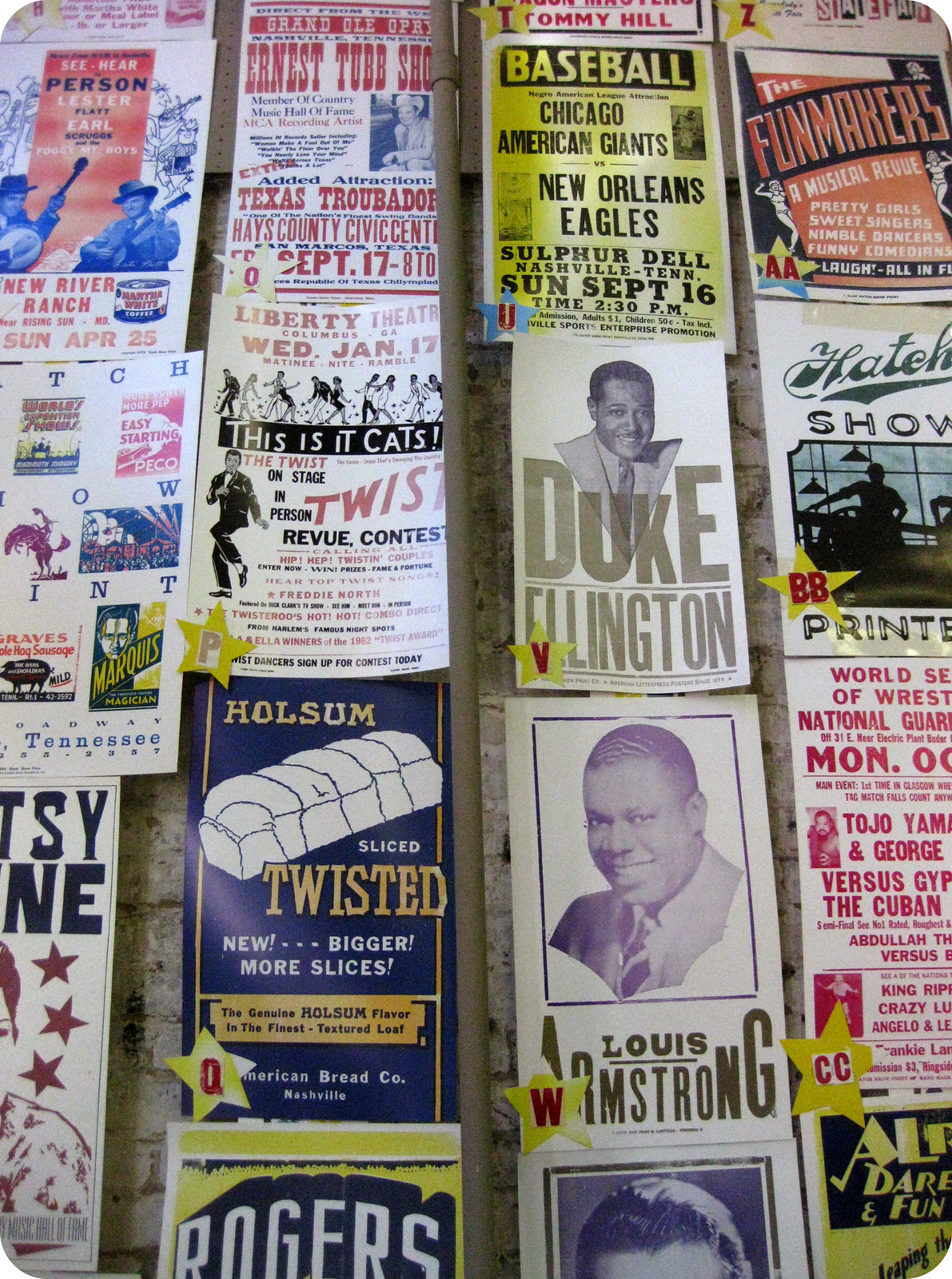The image captures a sprawling collection of vintage posters, advertisements, and handbills meticulously arranged in rows and columns on what appears to be a table. The assortment showcases a rich tapestry of cultural history, primarily featuring musicians, theatres, and sports events. Prominent among them are flyers for legendary performers, with names like Duke Ellington and Louis Armstrong standing out. One advertisement promotes "H-O-L-S-U-M, slice twisted, new, bigger, more slices," reflecting the era's commercial landscape. Another announces a show at the Liberty Theater on Wednesday, January 17th, with a lively proclamation, "This is it, cats." A baseball poster details a game between the Chicago American Giants and the New Orleans Eagles, highlighting the diverse subjects covered in the collection. There are also mentions of venues and events, such as New River Ranch and the Ernest Tubb Show, complete with images of musicians playing instruments, including men in cowboy hats. The entire scene evokes a strong sense of nostalgia, offering a vivid glimpse into past entertainment, sports, and advertising practices.